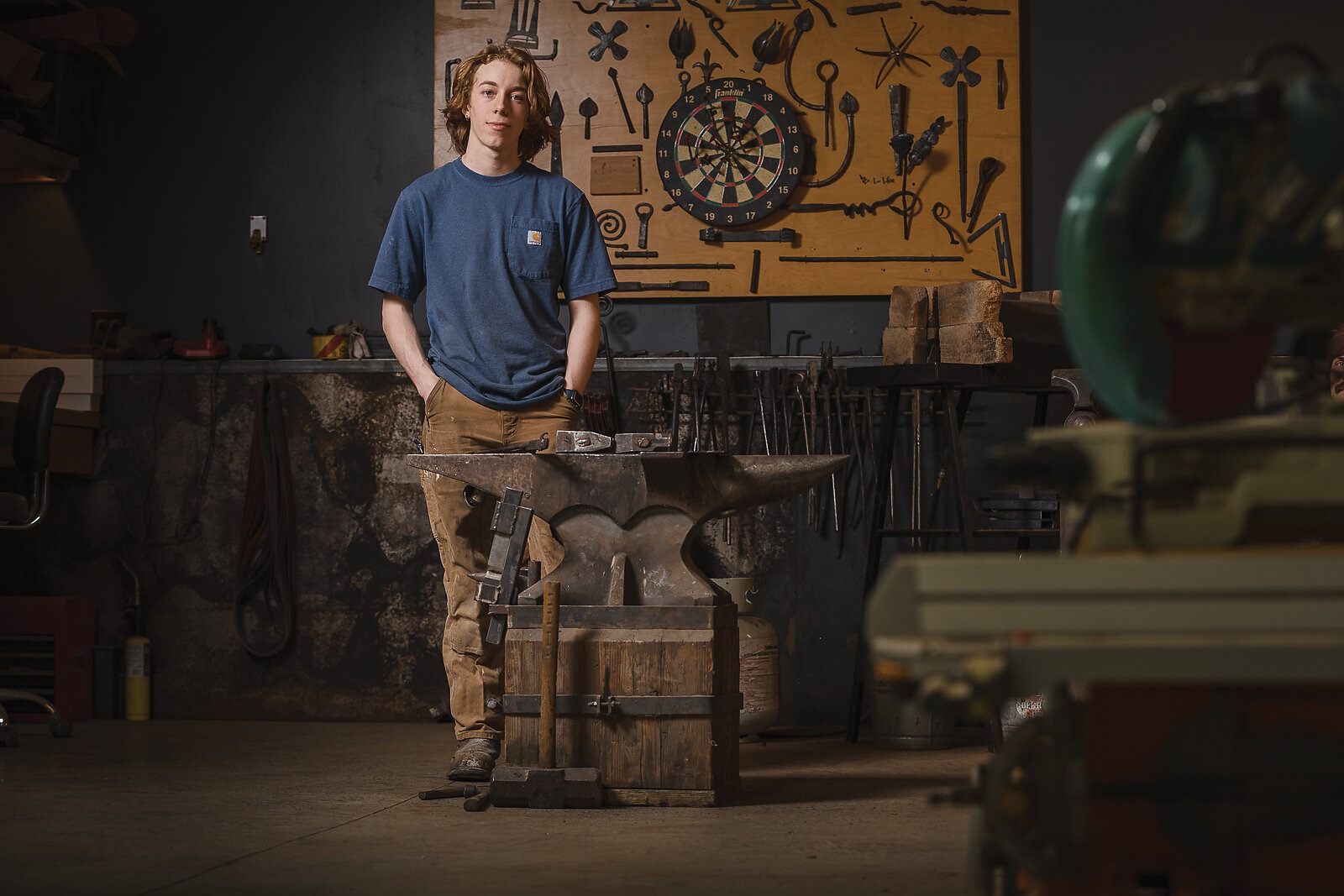The photograph captures a young man, likely in his early twenties, standing in a spacious workshop against a backdrop of a black-painted garage wall. He is positioned behind a prominent black cast iron anvil, which rests on a rectangular, wooden crate-like platform at the center of the image. The anvil, showing signs of rust with a blackish-brown hue, has two hammers placed atop it, and a large mallet lies on the floor in front. The man, wearing work pants and a blue t-shirt, stands casually with his hands in his pockets, smiling warmly. Behind him, a wall is filled with an assortment of tools, some mounted on a large wooden board alongside a dartboard, and others hanging from a shelf running the width of the wall. To the right of the scene, a substantial tool bench is visible, suggesting that the space is well-used for various projects and metalworking. Additional objects clutter the workshop, including a chair on a pedestal with wheels to the far left and a yellow cylinder topped with a nozzle. The workshop's floor appears to be brown concrete, adding to the industrial and utilitarian atmosphere.